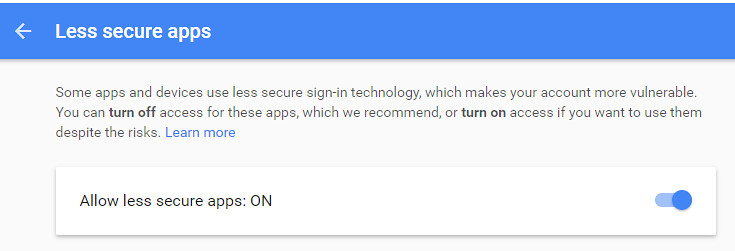This image is a horizontal screen capture, likely from a computer or tablet interface. Dominating the top portion is a prominent blue rectangle, extending across the full width of the image and labeled on the left side in white text with the phrase "Less secure apps" accompanied by an arrow pointing to the left.

Below this blue bar is a larger white rectangular section, which is slightly narrower than the blue bar above it. This section contains black text distributed across three rows, reading: "Some apps and devices use less secure sign-in technology, which makes your account more vulnerable. You can turn off access for these apps, which we recommend, or turn on access if you want to use them despite the risk." A "Learn more" link is highlighted in blue text towards the end of the message.

At the bottom of the white rectangle, there is a phrase in black text, "Allow less secure apps," followed by the word "ON" in all caps. To the right of this, a slide button with a blue dot is shown, indicating that it is toggled to the "ON" position within an oval-shaped slider.